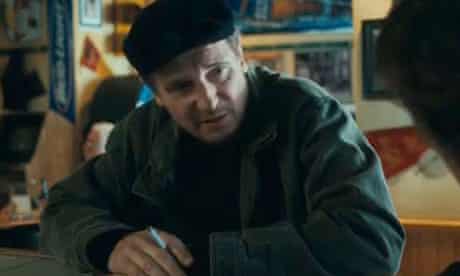The image appears to be a low-resolution, pixelated movie screenshot featuring the well-known actor Liam Neeson, who looks to be in his 50s or 60s. He is indoors, seated with his hands resting on a counter in front of him. Between the fingers of one hand, he is holding a white cigarette. Liam Neeson is dressed in a dark green, military-style jacket over a black long-sleeve shirt and wears a black cap. His face is turned slightly to the right, appearing to converse with someone whose face is mostly obscured but identifiable by dark hair. Behind him, the background features walls adorned with various designs, triangular flags, and photos, suggesting the setting could be a bar or related environment. There are also visible signs, including ones for Bud Light, adding to the bar-like atmosphere. The light from a right-side window softly illuminates Neeson's face, casting a somewhat stressed expression.